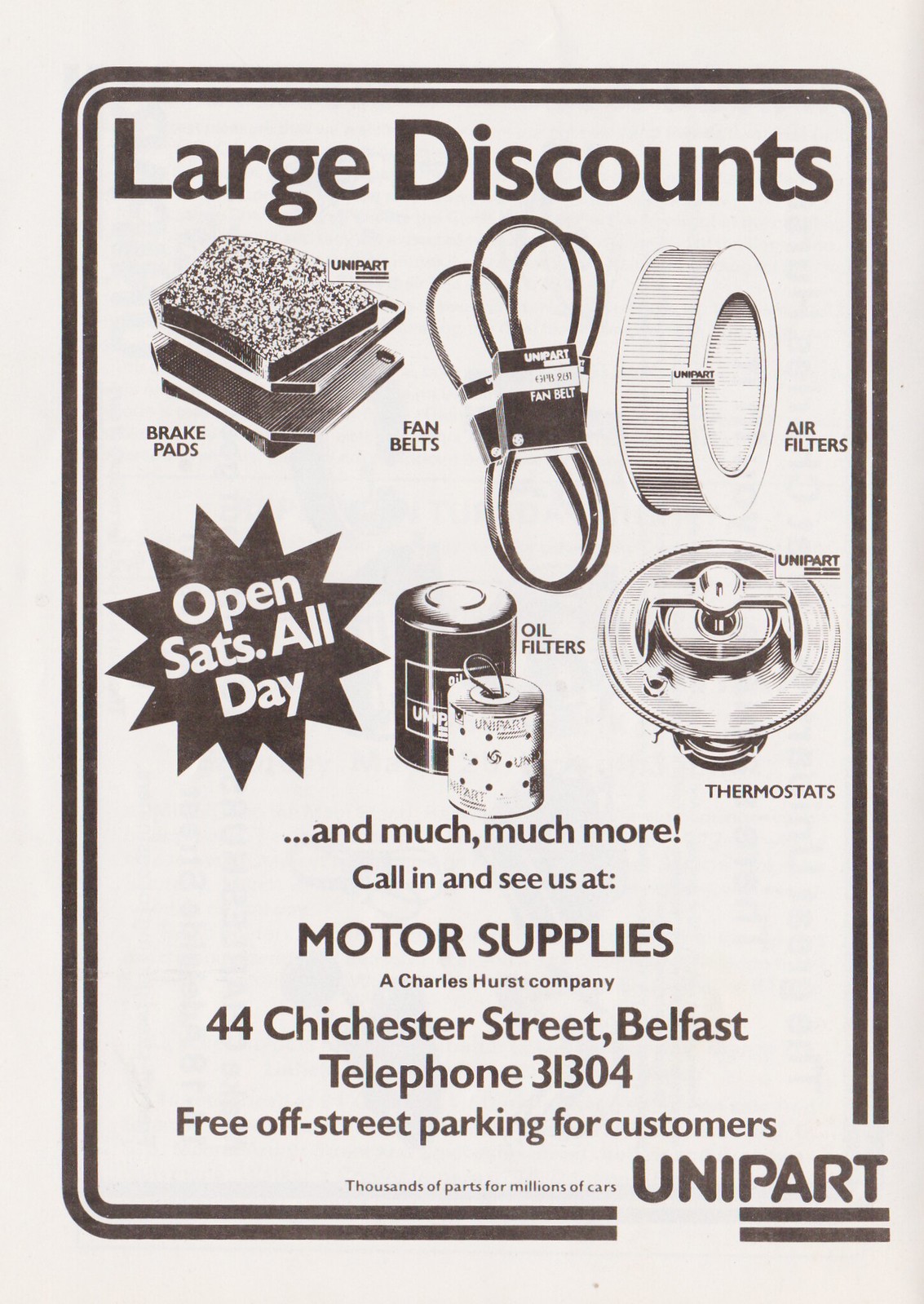This advertisement, likely from a magazine, features a black and white design set against a gray background. It is framed by a double black line border. At the top center, bold black letters announce "Large Discounts." The ad displays several black and white illustrations of car parts. From left to right, there are images of brake pads marked as "Brake Pads," fan belts labeled as "Fan Belts," a circular air filter with the caption "Air Filters," and a thermostat labeled "Thermostats." Near the bottom center, there are illustrations of two oil filters labeled "Oil Filters." Adjacent to these is a black star containing white text that reads "Open Sats All Day." Beneath this section, the ad promises "…and much, much more!" The text continues with a call to action: "Call in and see us at Motor Supplies, a Charles Hurst Company, 44 Chichester Street, Belfast. Phone 31304. Free off-street parking for customers." At the bottom center, bold text proclaims "Thousands of parts for millions of cars." In the bottom right corner, "Unipart" is prominently displayed in uppercase letters.